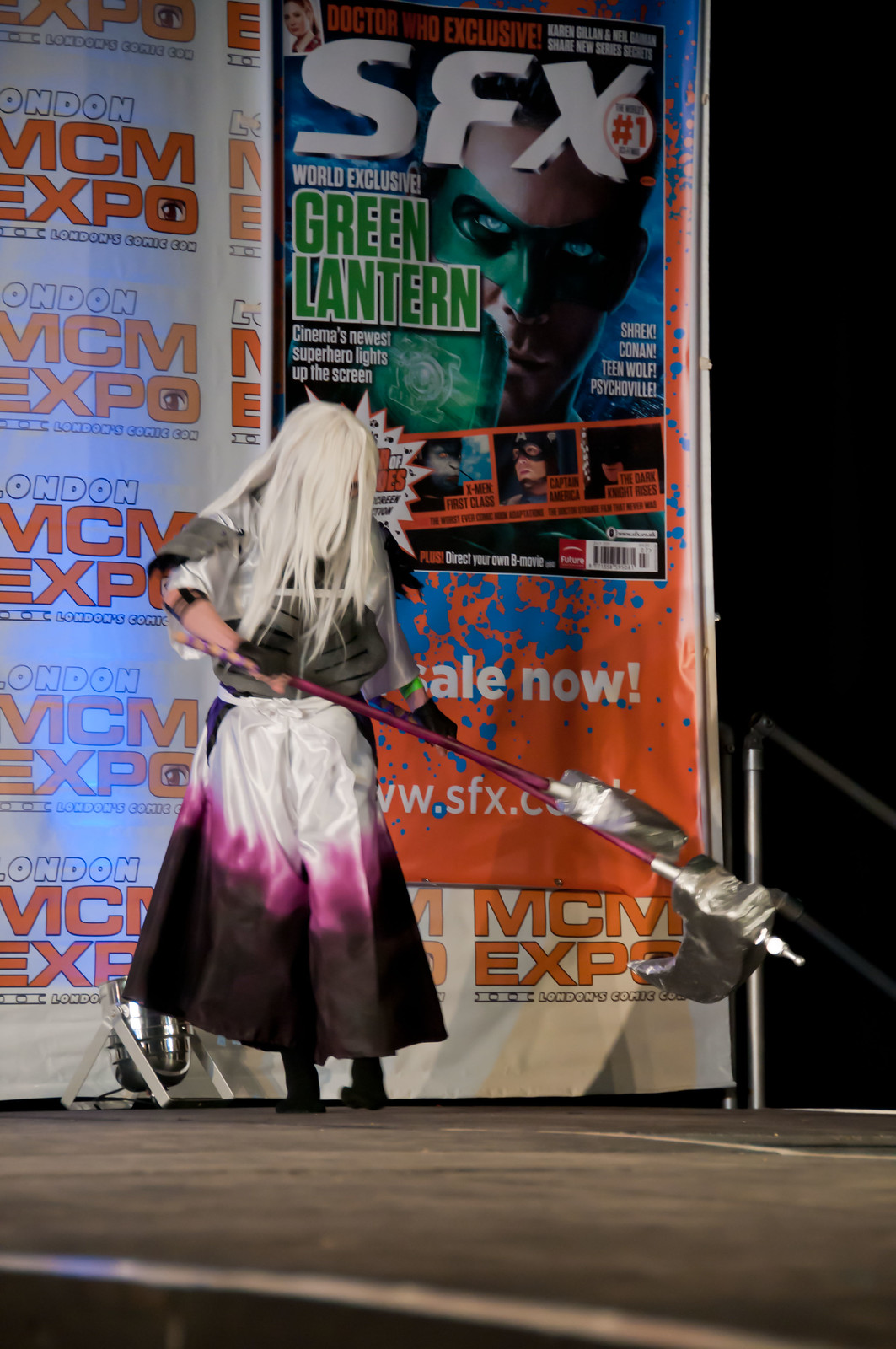A photograph captures a cosplayer performing at the London MCM Expo, evident from the prominent banner in the background. The individual, likely a young woman, is adorned in a striking costume featuring a long, white wig that obscures their face, and a dramatic skirt—dark at the bottom with a magenta swath, transitioning to white from the waist down. She wears a short-sleeve top that matches the gray-white hues of her hair. The cosplayer wields a pair of dual lances or spears with red handles and silver blades, adding a dynamic touch to her outfit. The scene is set on a stage with a black ground and a black scrim to the right. In the backdrop, an overlaying magazine cover for "SFX" highlights "Green Lantern," cinema's latest superhero, with vibrant orange, blue, green, and white colors.